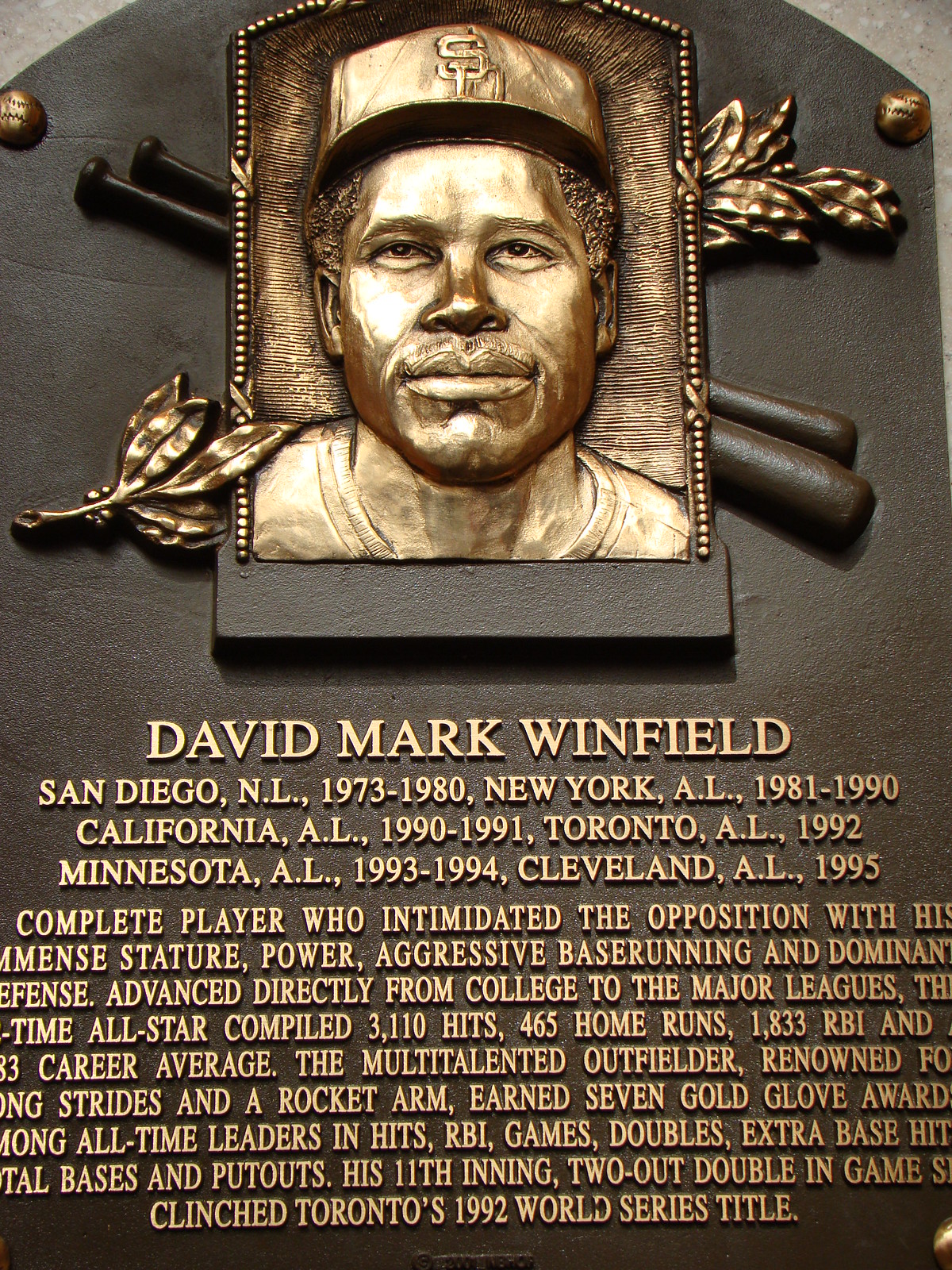The memorial plaque commemorates the legendary baseball player David Mark Winfield. Set against a dark metal background with shiny bronze accents, the plaque features a relief portrait of Winfield wearing a baseball cap with "SD," likely representing San Diego. Below the portrait, two crossed baseball bats and decorative leaves add to the plaque's ornate design. The text details Winfield's illustrious career, listing his tenure with various teams: San Diego NL (1973-1980), New York AL (1981-1990), California AL (1990-1991), Toronto AL (1992), Minnesota AL (1993-1994), and Cleveland AL (1995). 

Acclaimed as a complete player who intimidated the opposition with his immense stature, power, aggressive base running, and dominant defense, Winfield advanced directly from college to the major leagues. The plaque highlights his all-star career achievements, noting his 3,110 hits, 465 home runs, and 1,833 RBIs. Renowned for his long strides and rocket arm, Winfield earned seven Gold Glove Awards and is among the all-time leaders in hits, RBIs, games, doubles, extra-base hits, total bases, and putouts. A standout moment in his career, his 11th inning, two-out double in Game 6 of the 1992 World Series, clinched the title for Toronto. Some text on the plaque appears cut off, but its nine lines of accolades offer a testament to Winfield's exceptional contributions to baseball.